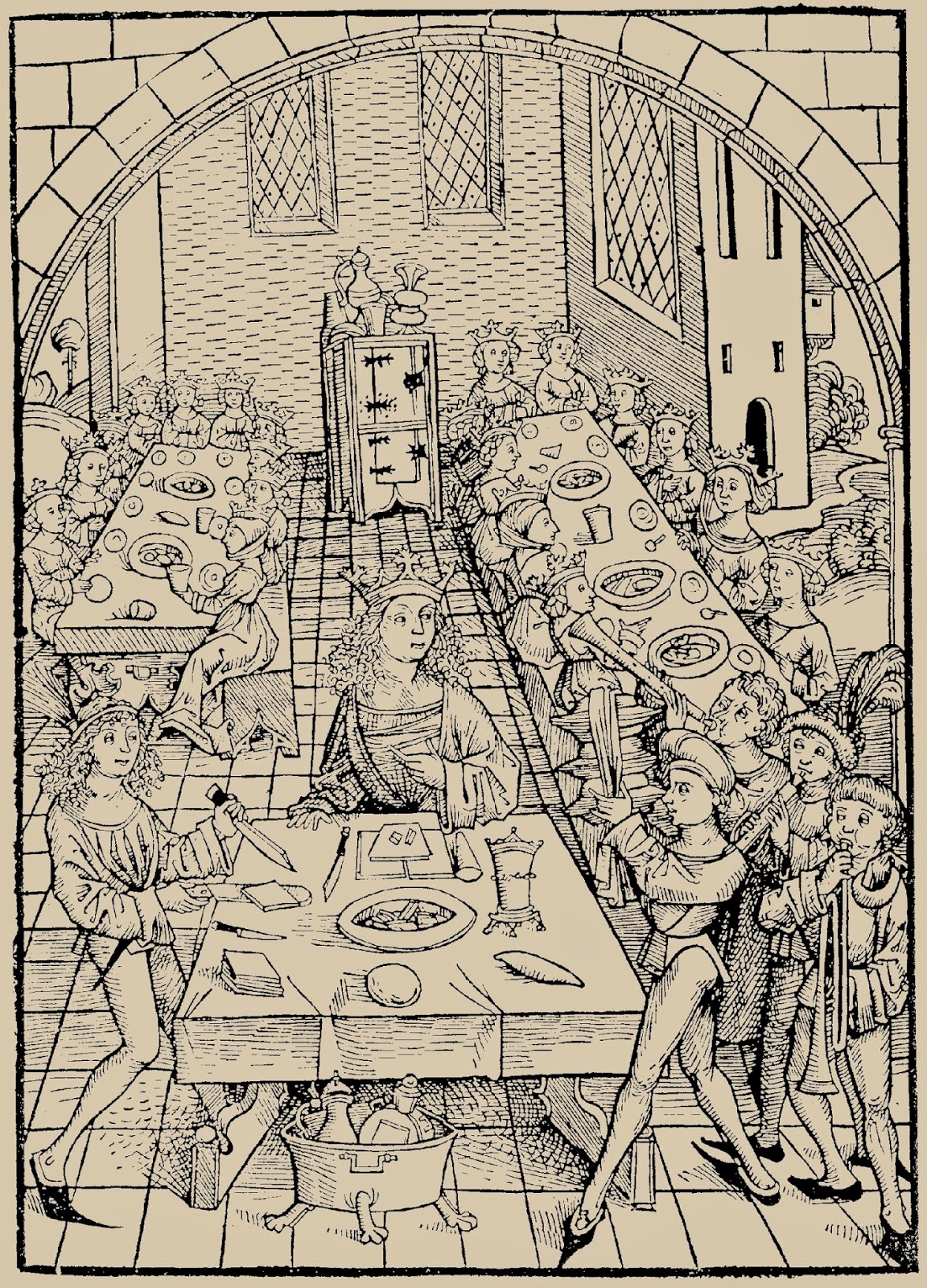This detailed, black-and-white drawing, set against a tan background, depicts an elaborate medieval feast inside an old-fashioned church or gathering hall. The scene is intricately rendered with black ink, showcasing a large room with an arched brick doorway at the top and rectangular tiled floors. The layout features three distinct tables: a square one at the front, a long rectangular table behind it, and another elongated rectangular table to the right.

At the forefront, a group of at least four musicians is playing instruments to entertain the diners. Among those seated at the front table, several individuals are adorned with crowns, suggesting their high status. A crowned lady appears to be the central figure, receiving special attention as food is being served to her, possibly cheese being cut by a servant.

The gathering scene reveals a majority of women seated and standing, with a few standing figures on the bottom right, indicating servants or attendants. The overall style suggests a hand-drawn piece or digitally created print, evoking a sense of medieval times through its detailed and historical ambiance.